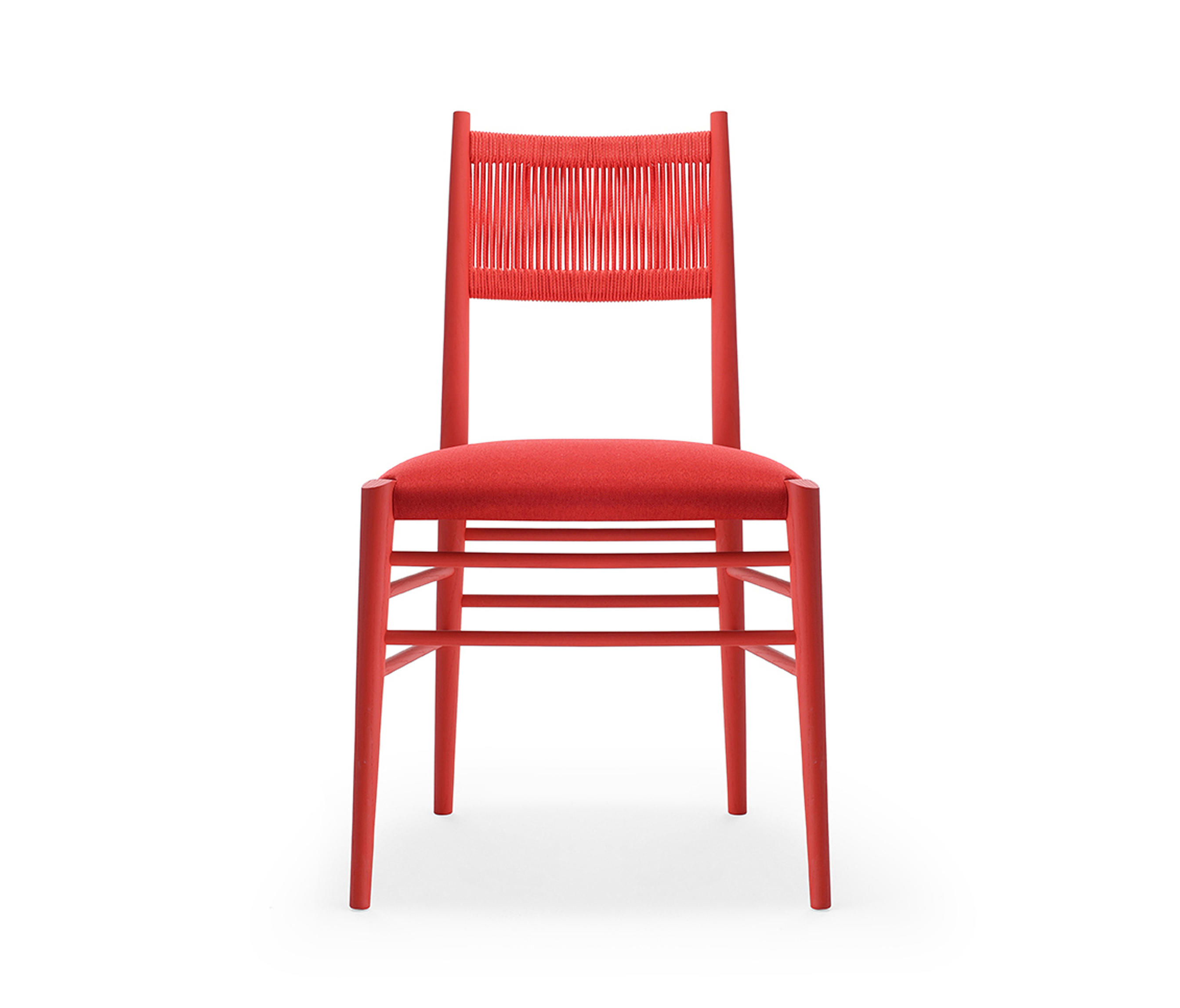This is a detailed image of a striking red chair set against a solid white background. The chair, viewed from the front, features a padded seat and a uniquely designed backrest. The backrest comprises two poles supporting a woven pattern made of wood, offering a blend of craftsmanship and simplicity, and it runs halfway down the back of the chair. The chair stands on four legs, each connected by two brace supports on the front, back, and sides, ensuring stability and strength. Additionally, a subtle black shadow is cast beneath the chair, grounding it in the pristine white setting. This combination of color and structure makes the chair a standout piece in the otherwise minimalist composition.